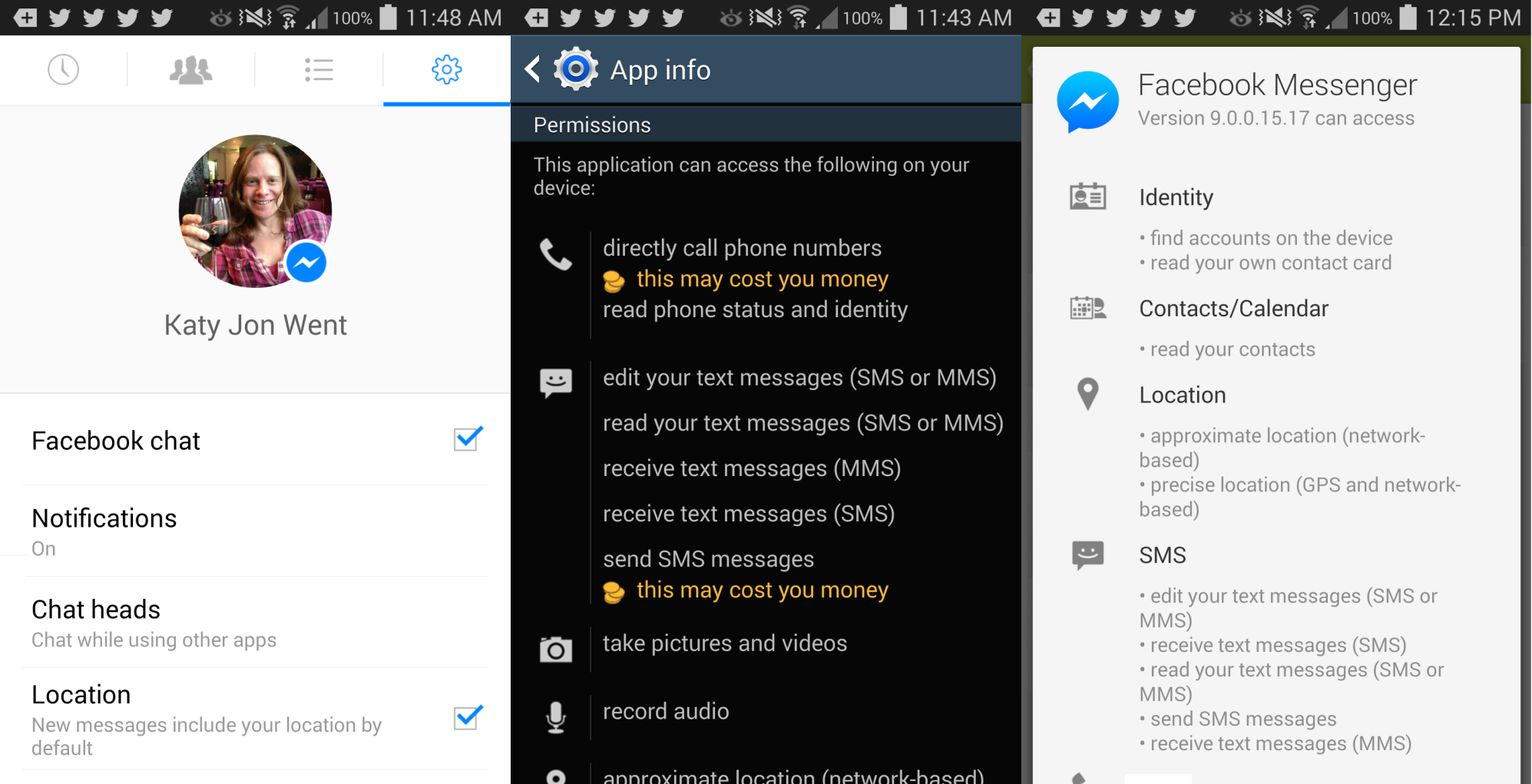In the left section of the image, there is a woman with short brown hair, holding what appears to be a bottle of alcohol or wine. Underneath her image, the name "Katie John Wendt" is displayed, spelled out as K-A-T-Y. Below her name, the text "Facebook chat" is visible, with a blue check mark inside a box to the right of it. Continuing down, the options "Notifications," "On," "Chat heads," and "Chat while using other apps" are listed, followed by "Location" with the note "New messages include your location by default." A blue check mark inside a box is also seen further to the right of these options.

Moving to the right side of the image, there is a black rectangle. At the top of this rectangle, an icon resembling a settings wheel is labeled "App Info." Below this, the heading "Permissions" is accompanied by an image of a phone and the text "Directly call phone numbers" in orange, with a warning "This may cost you money." Continuing downward, the phrase "This may cost you money" is repeated in orange next to another circular icon. On the right side, there is the text "Facebook Messenger" next to a blue circle with a horizontal line inside. Underneath "Facebook Messenger," the categories "Identity," "Contacts/Calendar," "Location," and "SMS" (in all capital letters) are listed.